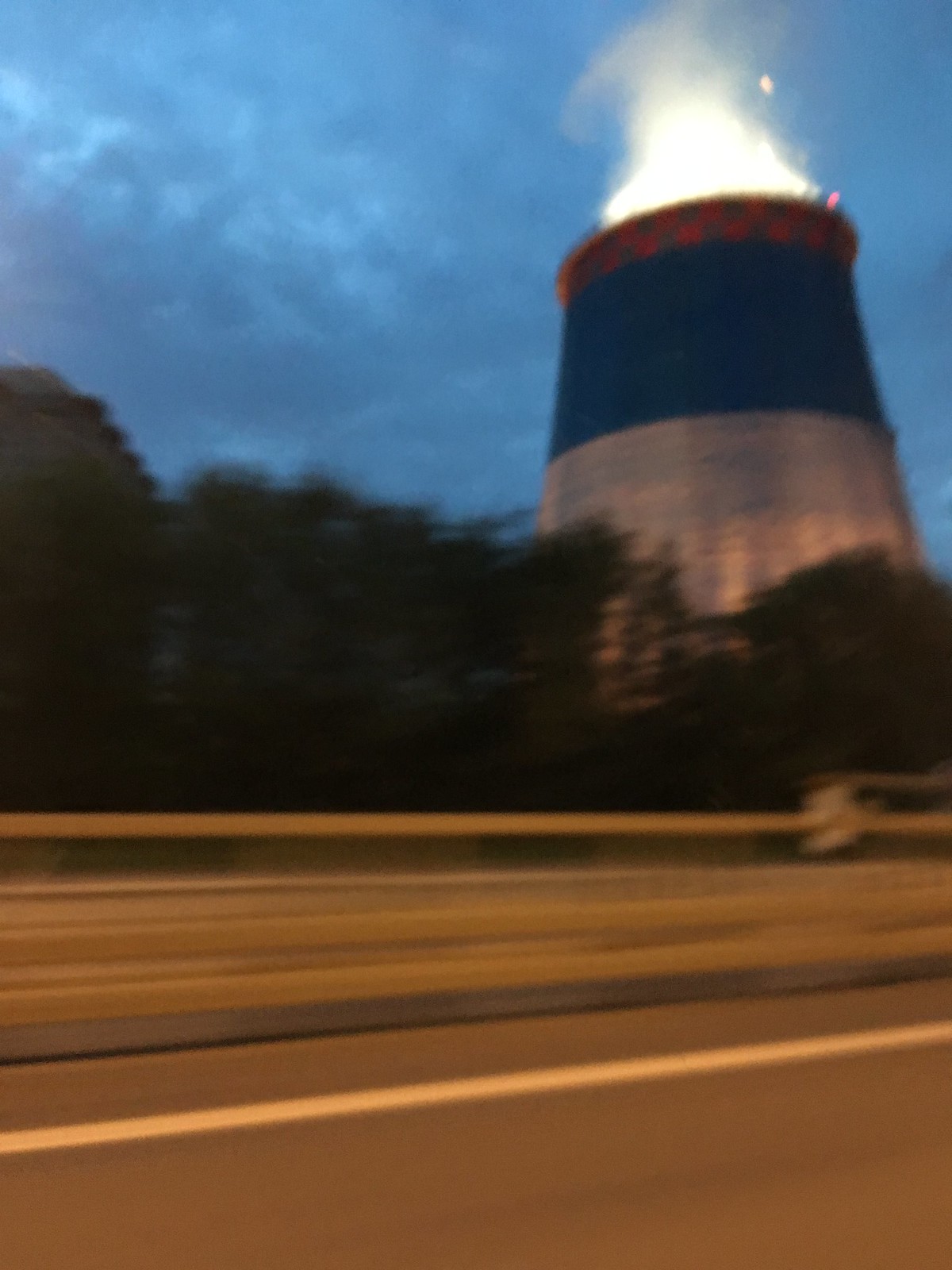This blurry photograph, likely taken from a moving car on a highway, captures the scene at nightfall as the sky transitions from blue to dark. Dominating the image is a large tower with a complex structure: the lower section appears metallic, the middle section is painted dark blue, and the top is capped with a red ring. The tower seems reminiscent of a nuclear reactor or water tower. At its top, a striking fire or intense light is visible, accompanied by plumes of white smoke. In the background, a row of silhouetted trees lines the other side of the road, with their dark forms contrasting against the dimming sky, creating an almost eerie silhouette. The highway surface is discernible, marked by a white stripe running alongside a guardrail, adding depth to the overall composition.